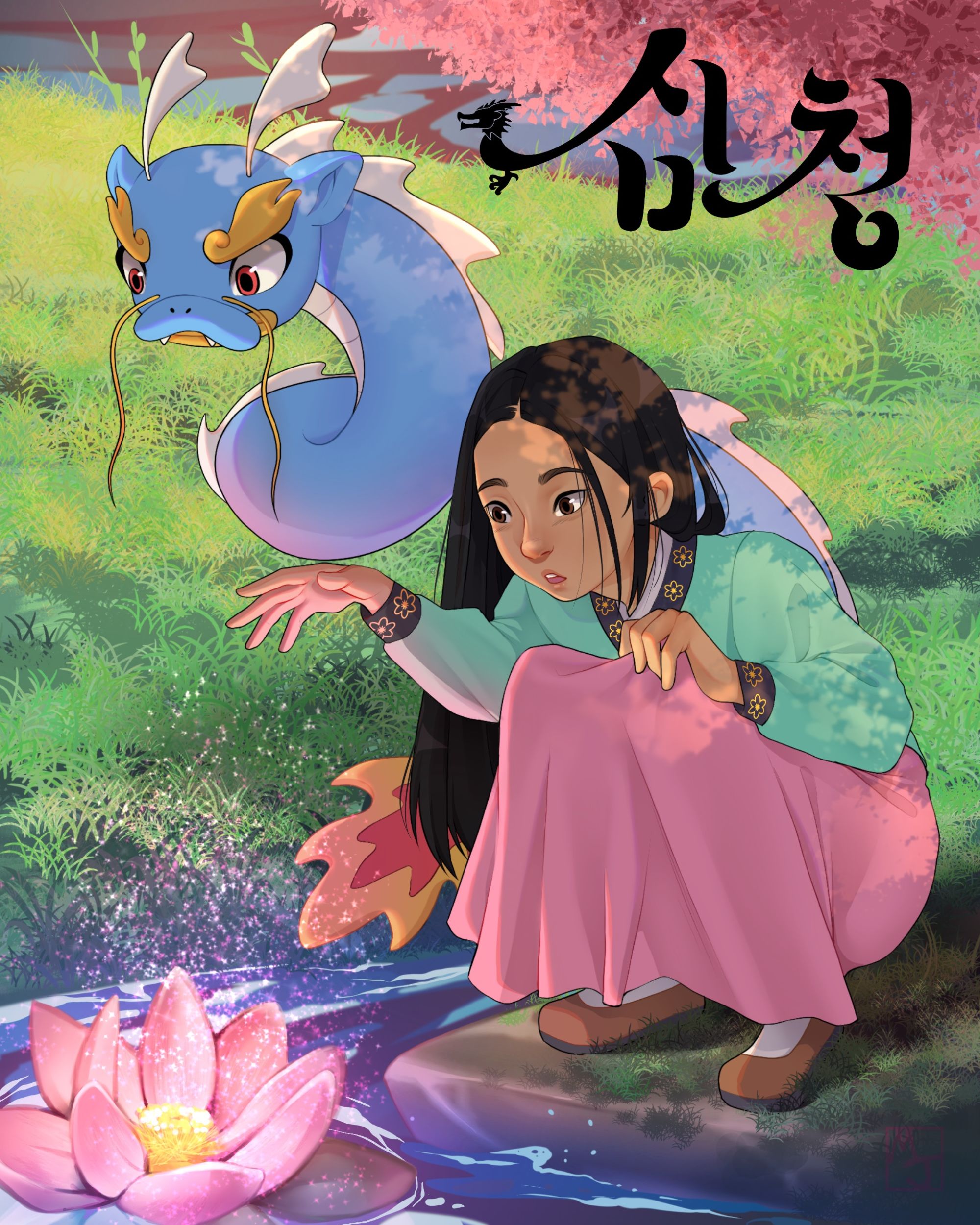In this vividly animated illustration, a young girl with long, dark hair and brown eyes is crouched by the edge of a serene pond. She is intently focusing on a large, radiant pink flower with a yellow center that captures her full attention. The girl is wearing a traditional outfit, consisting of a green top with black and yellow trim around the neck and sleeves, a long pink skirt, and rust-colored shoes. She also has white tights covering her legs.

Next to her, seated on the stone she is squatting on, is a friendly, bluish-purple dragon with pink ears, white fins, and scales. The dragon has golden eyebrows and little yellow catfish-like whiskers, lending it a mystical appearance. Its large size and gentle demeanor suggest it is her pet, reinforcing the magical aura of the scene. The background features a lush environment with green grass and a tree adorned with vibrant pink leaves, enhancing the fantasy atmosphere.

In the upper right-hand corner, there is stylized Asian writing, possibly Korean, integrated with a dragon-shaped design, further emphasizing the illustration's whimsical theme. The entire scene is bathed in a soft glow, with sparkling light emanating from the flower, adding an enchanting, almost dreamlike quality to the image.